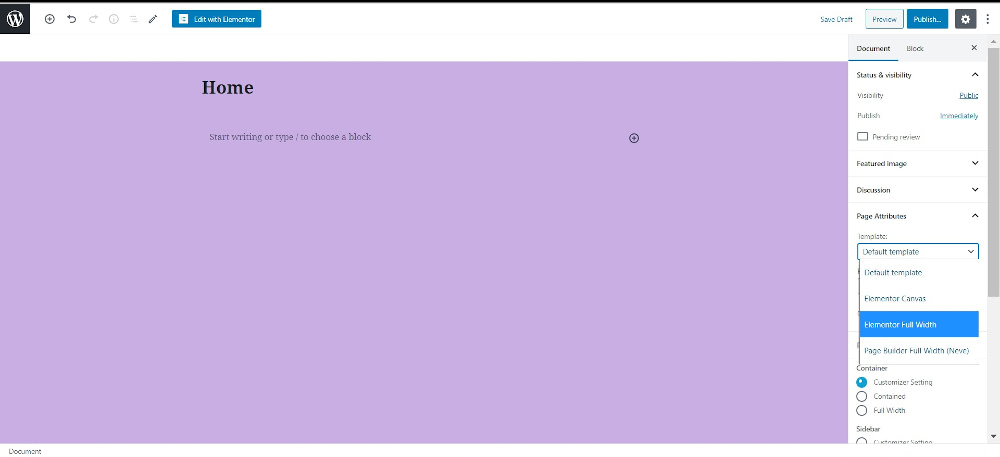This image depicts a miniature web page with a predominantly light purplish background that extends across most of the display, leaving a narrow white bar approximately an inch wide along the far right edge. At the top of the purplish section, "Home" is prominently displayed in black letters. Just below, a message reads, "Start writing or type / to choose a block."

In the upper left corner of the page, there is a logo featuring a plus sign within a circle, adjacent to a back arrow, a grayed-out forward arrow, an information (i) icon, and an edit button. Additionally, a teal rectangular box with unreadable text is present within this section.

To the right, along the white sidebar, a series of menu items are listed including "Status and Visibility," "Discussion," "Featured Image," "Page Attributes,” among others, providing various options to manage the content of the web page. The overall layout suggests a user interface for content creation or webpage editing.